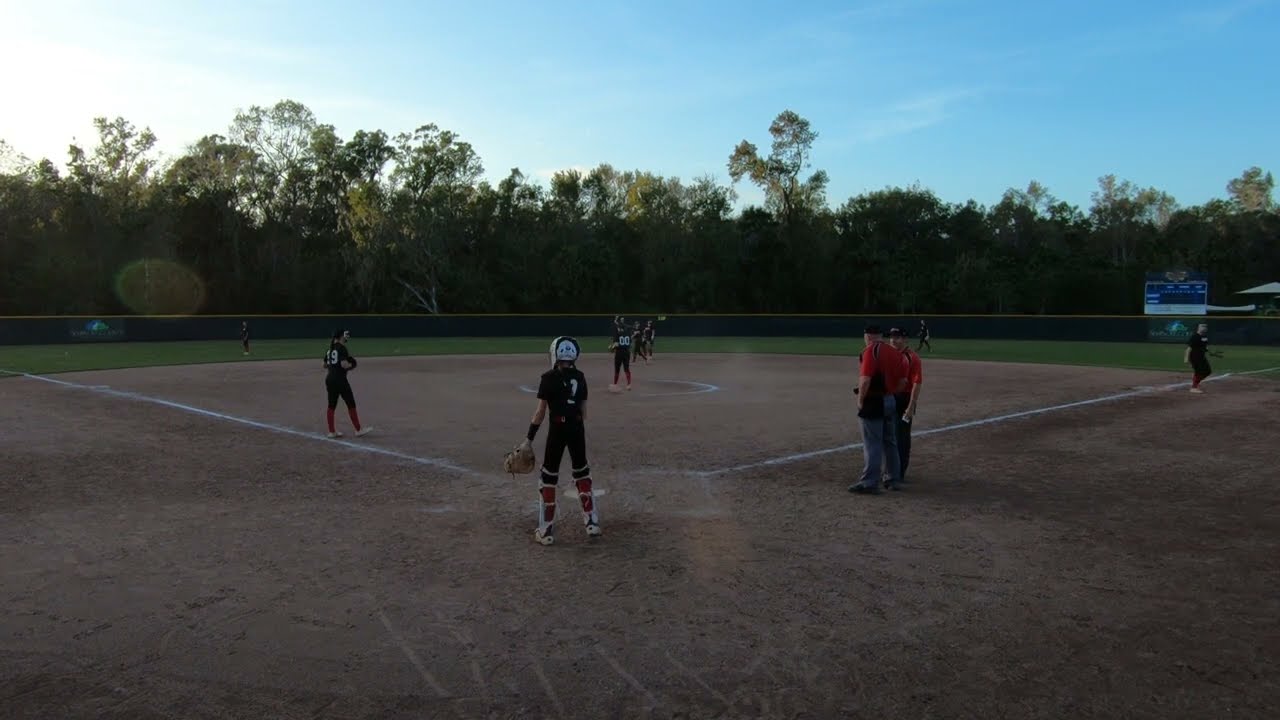This photograph captures a serene moment at a softball game from the vantage point behind the catcher. The players are paused in between plays, with the infield dirt grounds bathed in the gentle light of the setting sun, casting shadows across the field. The team, dressed in black uniforms accented by white numbers and red socks, is scattered across the field. The pitcher is poised on the mound, while the catcher stands and gazes outward. Several players are positioned near the bases and outfield, suggesting they are in a state of warm-up or anticipation for the next inning. Two umpires, identifiable by their red polo shirts and gray pants, stand near home plate. The outfield fence, highlighted by a distinct yellow line, separates the field from the dense tree line in the distance, hinting at the changing seasons with a sprinkle of leaves. Prominently, a blue scoreboard is visible to the right, just beyond the left-field fence. The field and the surrounding scene reflect a tranquil prelude to the game resuming.